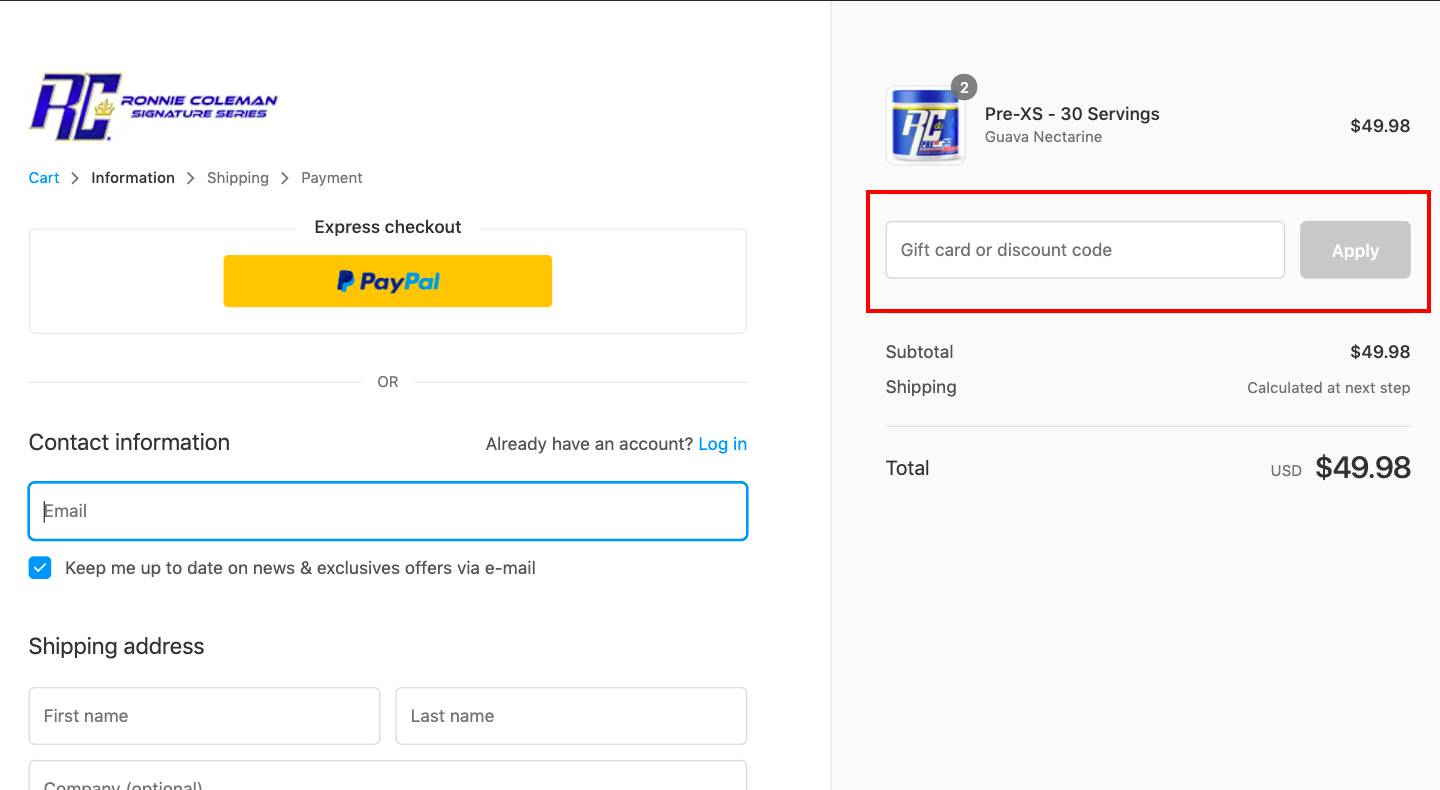Here's a detailed and cleaned-up caption for the image described:

---

The image is a comprehensive screenshot taken in portrait mode, likely from a laptop, displaying an online checkout process. At the top edge of the screen, spanning from the upper left-hand corner to the upper right-hand corner, there is a gray line. Below this line, the layout is divided into two columns.

In the left column, the top right corner features a logo of the Ronnie Coleman's Signature Series. Below the logo, there is a blue "In Cart" indicator followed by navigation options labeled "Information," "Shipping," and "Payment." 

Next, there's an "Express Checkout" section with an orange PayPal button prominently displayed. Below the PayPal option, a series of lines demarcated with "or" provide an alternative checkout method. Following this, the text "Contact Information" is visible, with a prompt on the right side saying "Already have an account? Blue login." A blue search bar is placed below, with a label "Email" and an option checked off in blue to "keep me up to date on news and exclusive offers via email."

The shipping section follows, requesting the user's address with fields for "First Name" and "Last Name."

In the right column, there is an image of the purchased product, indicating the Ronnie Coleman's Signature Series. The icon shows that two items have been selected. The product title "Pre-Excess 30 Servings Guava Nectarine" is displayed along with the total price of $49.98, which equals approximately $25 per item.

A red box highlights the "Gift card or discount card" entry field, beside which is a gray "Apply" button for entering a promotional code. The subtotal is listed as $49.98, with a note that shipping will be calculated at the next step. The total amount due currently stands at $49.98, and the prompt encourages the user to enter a gift card or discount code to reduce the total cost.

---